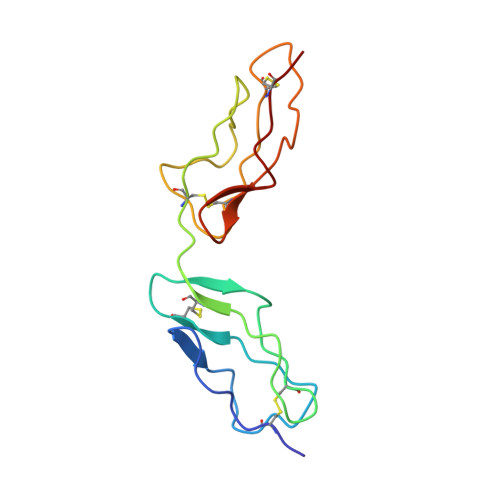The image features an intricate array of interconnected, colorful squiggly lines set against a pure white background. Dominating the top half, a swirly orange line morphs into a bird-like shape on the upper right, enclosing a bright red line that zigzags towards the center and transforms into a twisted red arrow. Adjacent to this, a twisting lime green line merges with yellow, descending towards the center and blending into orange, ultimately attaching itself to the tip of the red arrow.

Below this central cluster, another grouping unfolds. A teal arrow, pointing right, evolves into a teal squiggly line that journeys down to the bottom right corner of the image. Positioned under this, a lime green rectangle connects with the lime green line from above, transitioning into a line that also flows to the bottom right. An aqua blue twisted rectangle, linked to the teal arrow, transitions into an aqua line that similarly heads downward and right. Further below, a bluish-purple arrow points down and right, leading into a bluish squiggly line that continues to the bottom right.

The drawing is a vibrant tapestry of colors—blue, red, teal, green, orange, yellow—interweaving and connecting in various complex ways, reminiscent of a spontaneous, abstract squiggle drawing. It could depict a scientific or electronic diagram, illustrating interconnections that are not immediately apparent. The overall impression is one of whimsy and complexity, as if someone took colorful pens and freely drew interconnected lines that dance across the canvas.